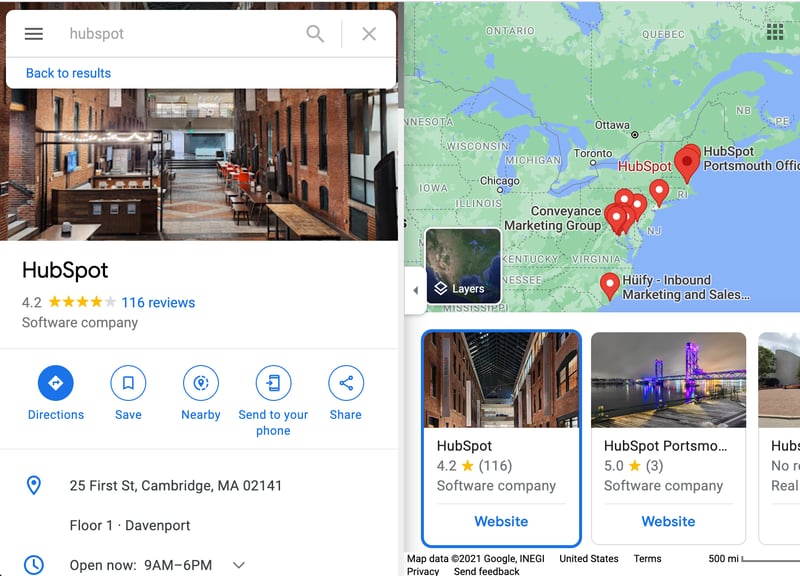This detailed image captures a search result for HubSpot, highlighting a range of relevant information and visual elements. At the top, the interface offers a "Back to Results" option, followed by an image of a long hallway featuring steps descending to a lower area, elegant benches, and a beautifully adorned floor with a diamond pattern. HubSpot is listed with a rating of 4.2 out of 5, based on 116 reviews, categorizing it as a software company. The interface includes interactive circles for actions such as getting directions, saving the location, sending it to your phone, and sharing it.

The address for HubSpot is displayed as 25 First Street, Cambridge, Massachusetts, 02141, located on the first floor of the Davenport building. The business hours are indicated with a clock symbol, showing that it is currently open from 9 a.m. to 6 p.m., accompanied by a downward arrow.

To the right of the main details, there is a map featuring various pins along the East Coast of the United States, marking different locations. One location is labeled "Huffy Inbound Marketing and Sales." The overall information reiterates HubSpot's rating, review count, and classification as a software company, with additional details extending further to the right.